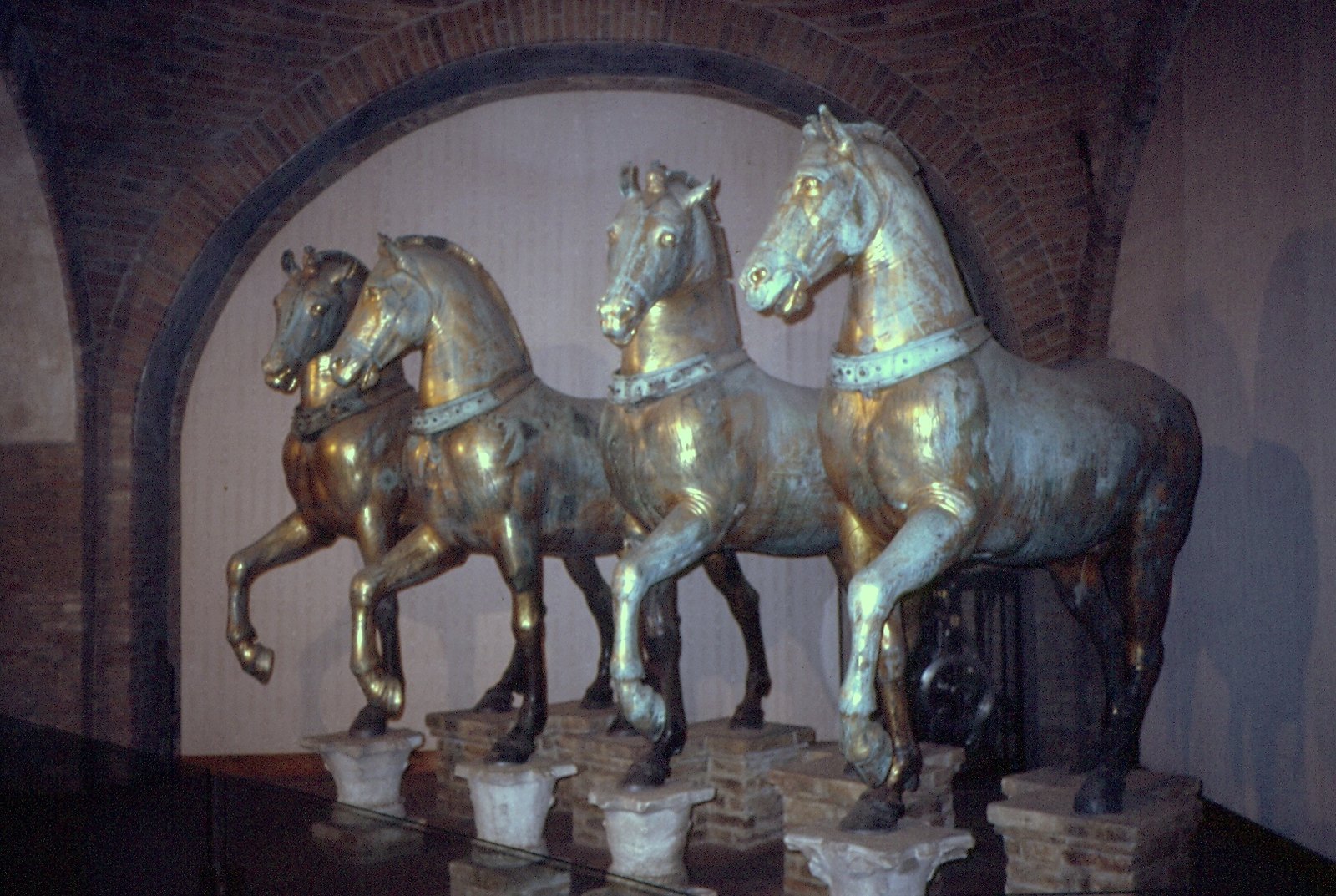This color photograph captures an interior setting featuring a display of four life-size bronze horse statues, each with a patina that gives them a partially gold appearance, though some of the gold looks worn off. These statues are positioned with one of their front legs raised, mimicking a prancing or mid-gait stance. The horses stand on individual brick pedestals in the foreground, located near the left corner of the image, within a glass enclosure or behind a glass partition. In the background, a partially walled-off arched brick doorway is visible, adorned with some wooden boards. The surrounding wall is white, interspersed with red brick sections and an awning-like structure, providing a contrasting backdrop to the bronze figures. The overall scene is one of stark focus on the detailed equine sculptures, devoid of other distractions.